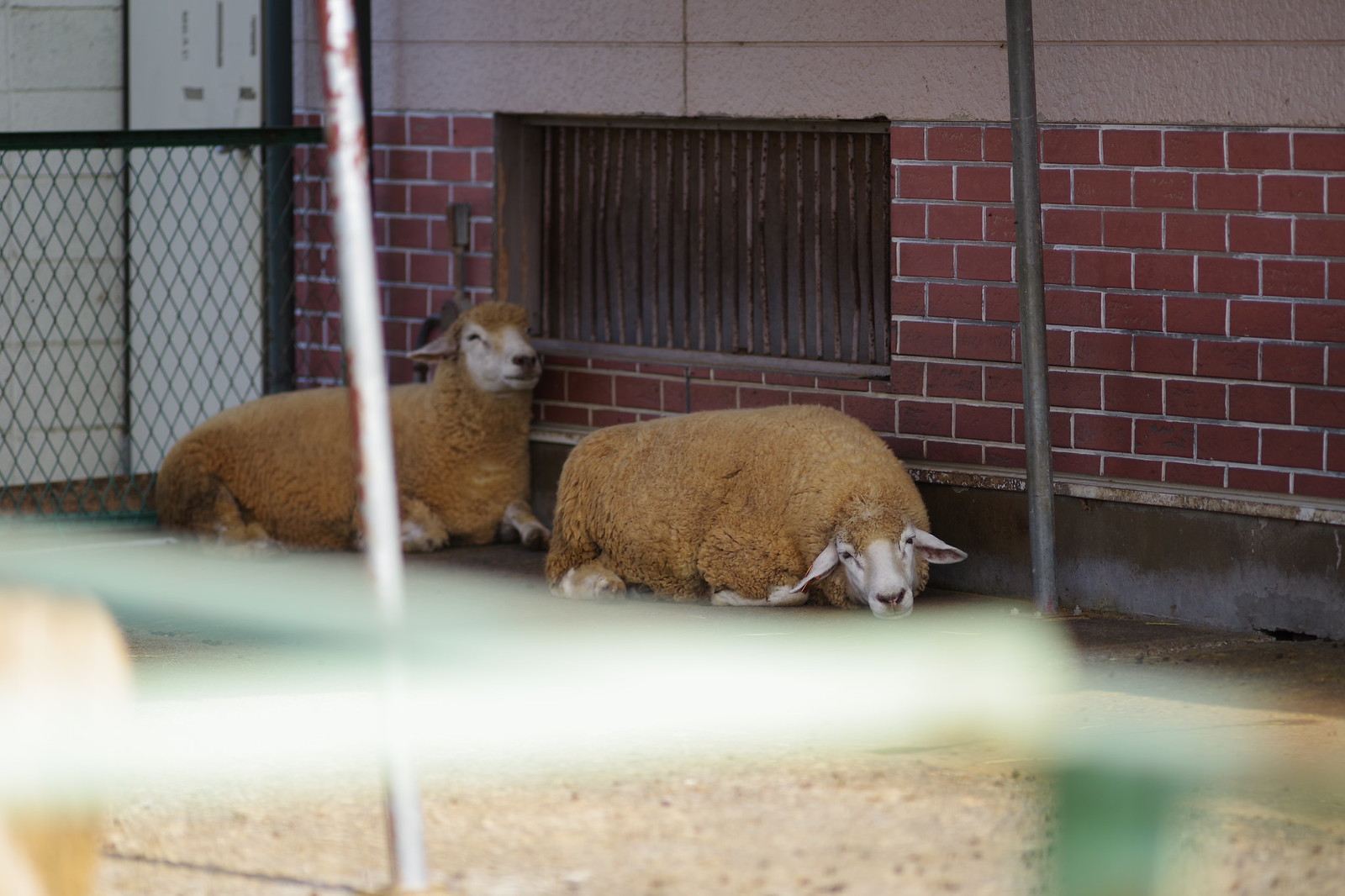This detailed photograph captures two sheep lying in an enclosure. The surroundings consist of a textured surface that appears to be sand or stone. The sheep are positioned against a red brick wall adorned with a central gray grate, with a distinctive upper section of white, textured plaster, suggesting the enclosure is outdoors. In the foreground, a green and white blurred structure, likely a guardrail or part of a fence, obscures some details. A silver pole with red-flecked paint is visible near the sheep. One sheep rests with its head on the ground while the other has its head raised, partially in front of the grate. Their wool is a unique brownish-orange, contrasting with their white faces and legs. Despite their woolly appearance, both sheep look notably plump. The overall atmosphere, enhanced by the various described elements, suggests a somewhat neglected or somber zoo-like environment.